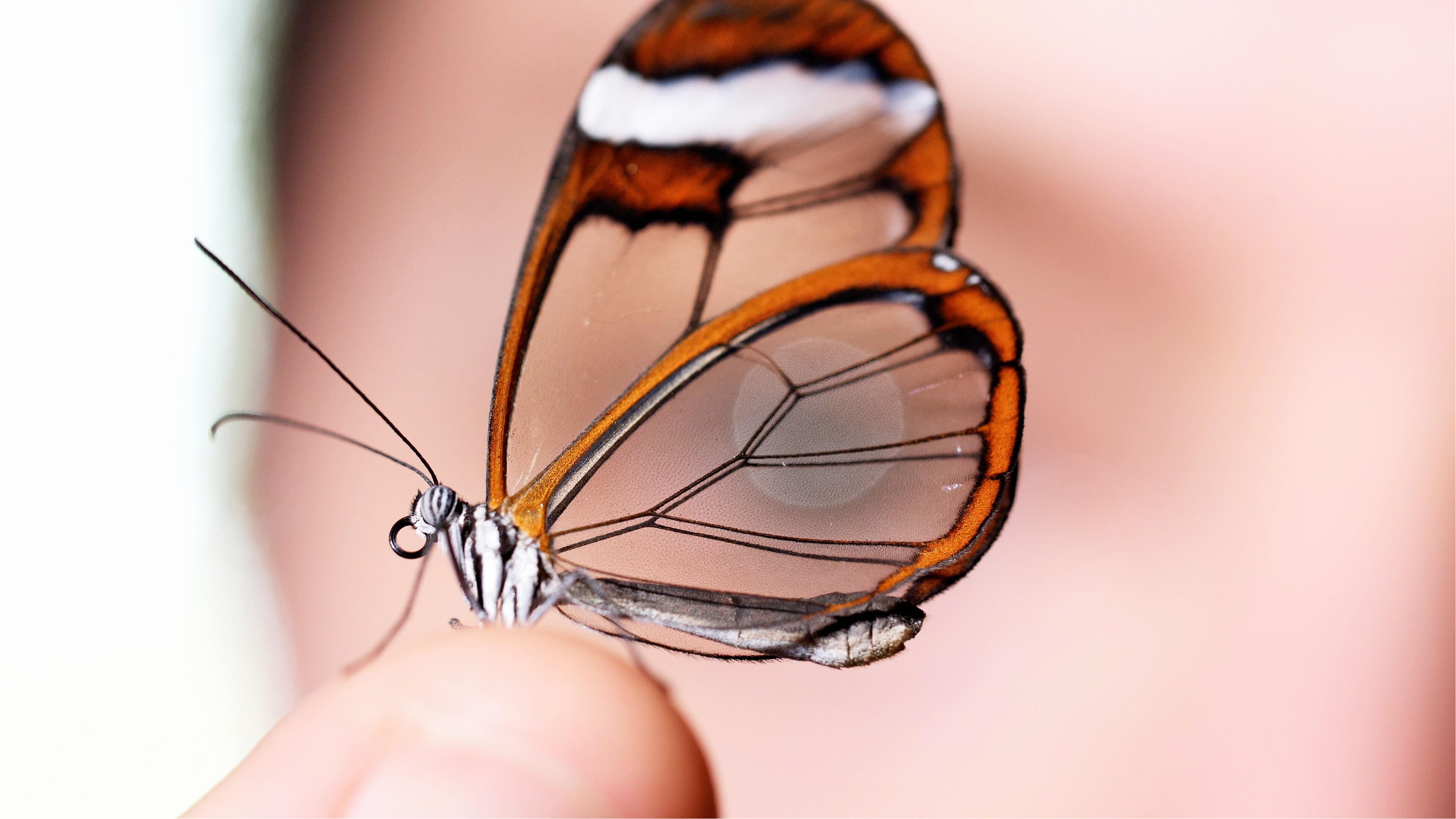In this detailed photo, a delicate butterfly with translucent wings perched gracefully on a person's finger takes center stage. The person's face forms the blurred background, with an eye and eyebrow faintly visible through the clear sections of the butterfly's wings. The butterfly displays a striking combination of colors and patterns: its wings have a brown and orange border, accented with fine black lines, and sections of bright white and orange near the top. The main body of the butterfly is striped in black and white, with its legs in white and its long, black antennae extending prominently. The wings' transparency beautifully reveals the blurred details behind them, creating a captivating juxtaposition of sharp foreground and soft background.